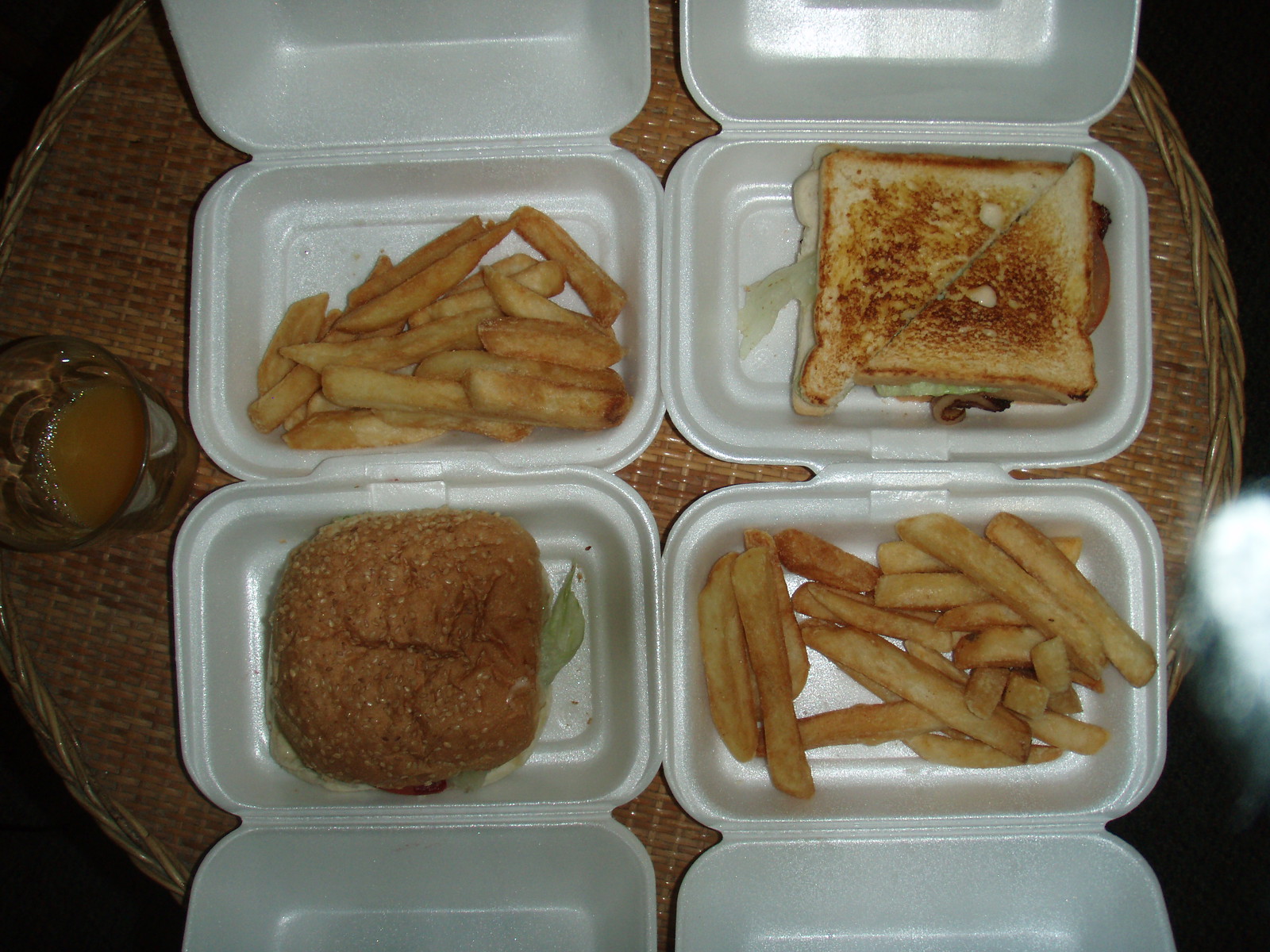This aerial photo captures four rectangular, polystyrene foam take-out boxes with hinged lids, all open to reveal their contents. Arranged on a round wicker table, the boxes are positioned with their lids unanimously directed outwards, ensuring the food is visible. In the upper left-hand and lower right-hand boxes, thick-cut french fries are neatly piled. The upper right-hand box contains a diagonally-cut sandwich on grilled, toast-like bread, with bits of lettuce and possibly mushrooms or grilled onions peeking out. The lower left-hand box holds a burger on a seeded bun with lettuce visible around its sides. Accompanying the food, a glass with some sort of liquid sits on the left side of the table, and a decorative porcelain object in brown adds a touch of elegance to the scene.